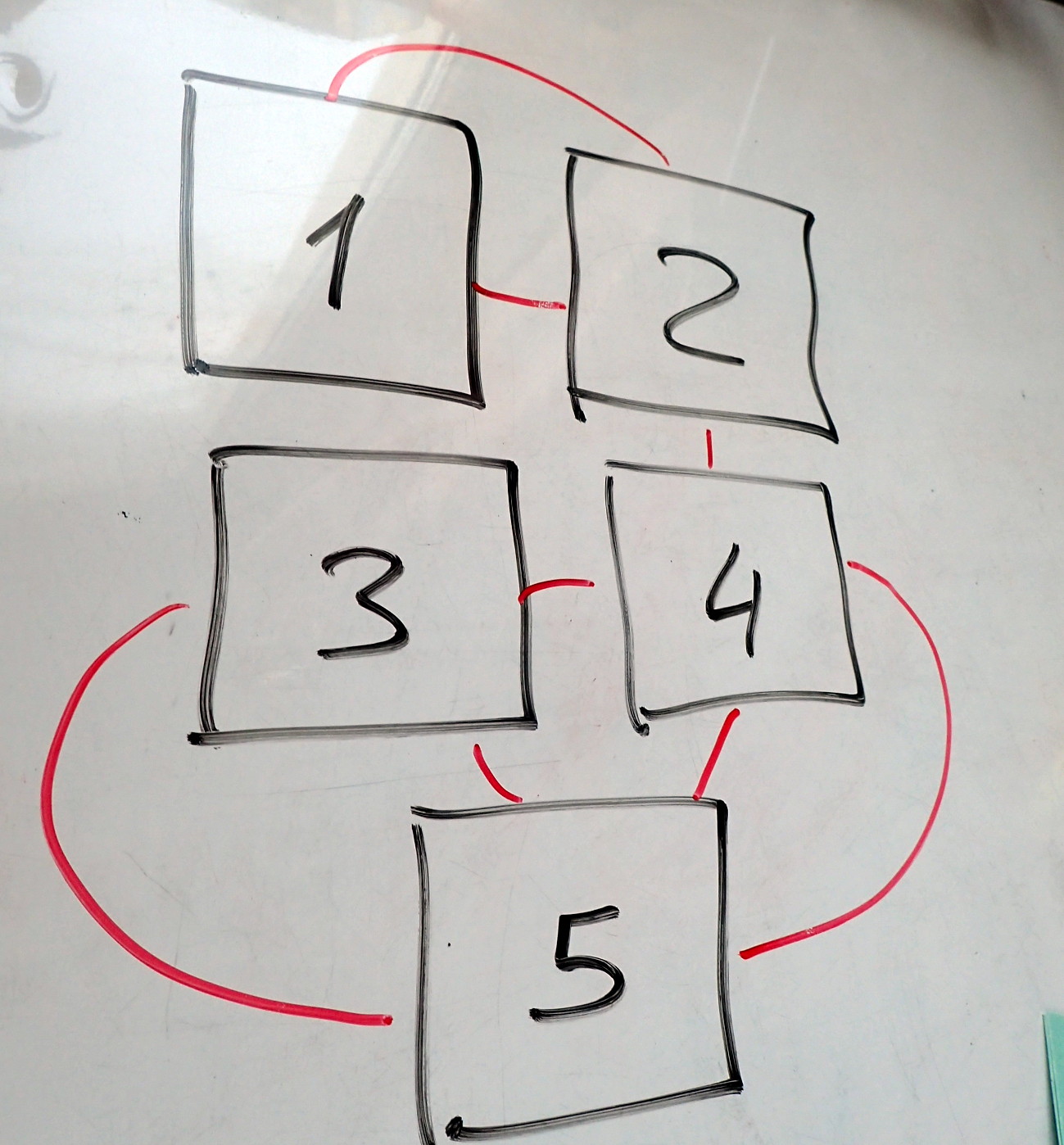This image features a loosely drawn flowchart or diagram on a whiteboard, depicted with various red lines connecting numbered boxes. The photograph is taken from a front angle, slightly skewed to the right, making the left side appear marginally closer. A noticeable glare from the room's light source is visible in the top left corner of the whiteboard.

At the very bottom of the diagram, there is a square with the number "5" inside. From this square, two broad red lines curve upwards, leading to boxes labeled "3" (top left) and "4" (top right). Directly above these boxes, there are smaller red lines extending vertically to connect to them. A short red line horizontally connects the tops of the "3" and "4" boxes.

Further above, on the top left and right respectively, are the boxes labeled "1" and "2." A red line arcs over from "1" to "2," and another direct red line connects "2" to "4." The lines and boxes are generally rough and inconsistently drawn, with some corners overlapping and the box for "5" being incomplete at the bottom left.

The whiteboard itself is relatively clean, with just a few smudges scattering its surface. The overall structure of the diagram is basic, with no elaborate embellishments or additional annotations.